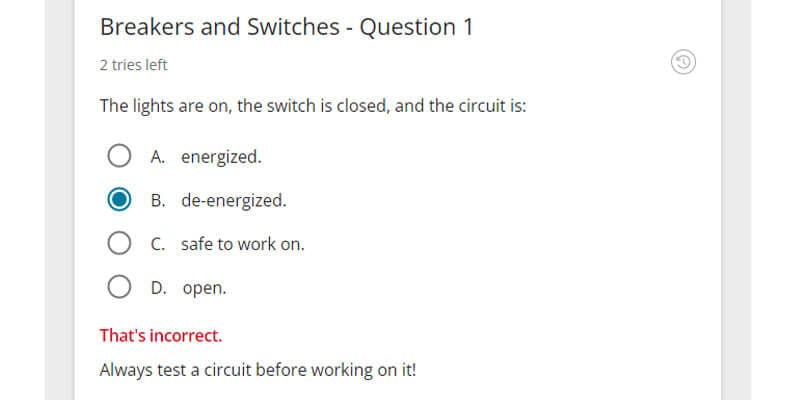The image shows a screen capture featuring a multiple-choice question interface. At the top of the screen, the heading "Breakers and Switches" appears in black text against a white background. Beneath this, the text "Question One" is displayed, and a smaller gray text underneath indicates, "Two tries left."

The actual question, written in black text on the white background, reads: "The lights are on, the switch is closed and the circuit is:"

- Option A: Energized
- Option B: De-energized
- Option C: Safe to work on
- Option D: Open

Option B has been selected, as indicated by a green and white circle to the left of it. Below the options, the text "That's incorrect" is written in red. Further down, a reminder in black text states, "Always test a circuit before working on it."